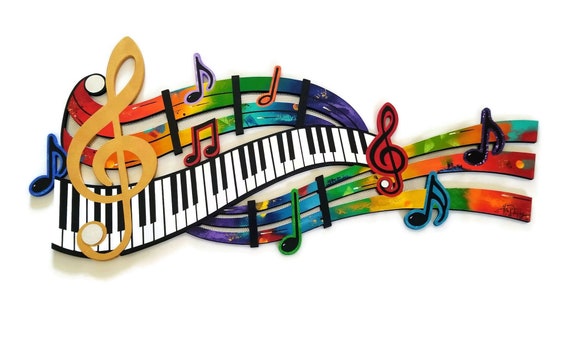This is a rectangular, computer-generated painting of piano keys and musical notes, rendered in vibrant, eye-catching colors. The central subject is a keyboard that appears to be curved and bent, creating a deliberately unrealistic yet visually appealing look. The keyboard, which includes all major, minor, flats, and sharps keys, winds dynamically from the left to the right across the white background.

Above the keyboard, there are rainbow-colored musical bars that stretch from the left side of the painting, overlayed with various musical notes and symbols. These include ampersand-like shapes, treble clefs, and traditional musical notes, some of which are placed on lines indicating their pitch.

A striking feature of the painting is a giant gold musical note placed slightly off-center towards the left. Surrounding it are several other colorful notes: a purple one, a red double note, and a pinkish note. Below this colorful cluster, the piano keys stretch across the canvas with fewer black keys positioned towards the top.

The piece also showcases three additional lines of music notes that emerge from under the piano keys, extending left to right. These lines and notes are a mix of colors—purple, yellow, red, blue, green, orange—with red-tipped ends. Prominent among these is a green note immediately beneath the keyboard, a large red note at the end of the keyboard, a black note with a blue border slightly down and to the right of that, and a nearly black note towards the far right end of the image.

A black border frames the entire scene, adding a finishing touch to this vibrant and dynamic musical composition that almost appears as a real object.